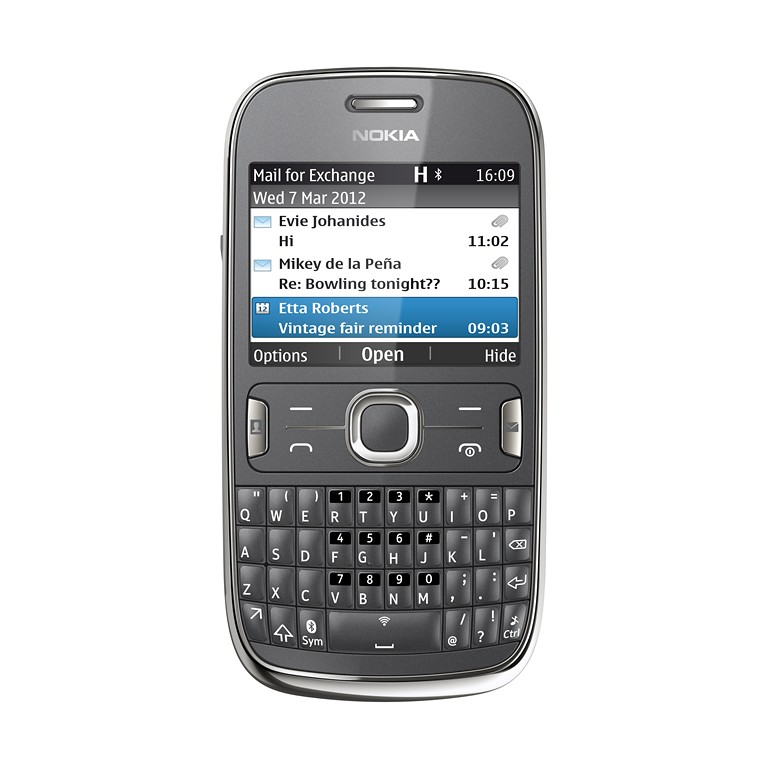A detailed and cleaned-up descriptive caption for the given image could be:

"This image showcases an old Nokia phone, specifically the Nokia 1600 model. The screen displays a scene dated Wednesday, March 7, 2012, capturing a snapshot from over a decade ago. The phone's interface shows several text messages, highlighted by a conversation from Evie Jonas to Mike de la Pena, discussing plans for bowling at a place called Robbers, which appears to be a vintage-themed bar. The phone screen also features some emails, indicated by the mail icon at the top. This nostalgic image offers a glimpse into the communication technology and social interactions of the early 2010s."